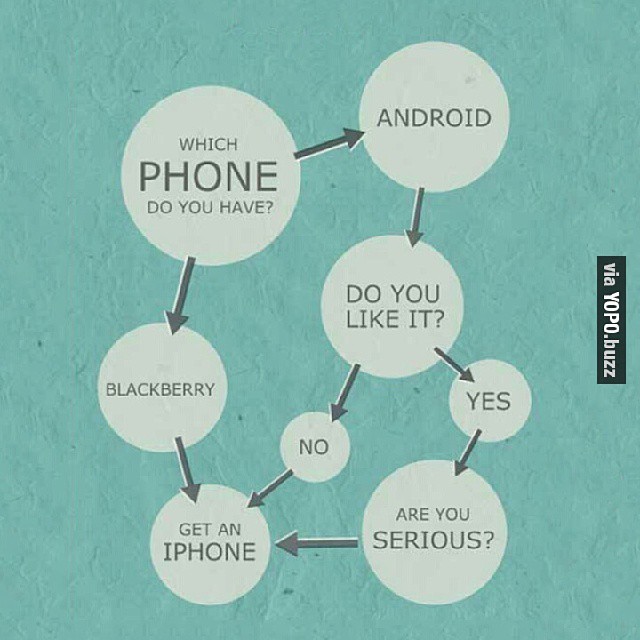The image is a detailed infographic designed with a satirical tone, likely intended for social media sharing. The infographic features a teal blue, textured background resembling poorly applied paint on drywall, and at its center, a network of pale-colored circular disks connected by arrows forms a flowchart. This flowchart, which humorously guides viewers towards purchasing an iPhone, includes various pathways based on different user responses. The main circle at the top asks, "Which phone do you have?" with two branches leading to "Android" and "BlackBerry." If you follow "Android," the flowchart further questions, "Do you like it?" leading to either "No" or "Yes," both of which point to "Get an iPhone." Similarly, selecting "BlackBerry" leads directly to "Get an iPhone." The arrows and disks predominantly use black text on a green and gray color palette. To the right-hand side, there's a black panel indicating "via Yopo.buzz," adding a layer of credibility or attribution to the image. Throughout the diagram, the humorous intent is clear, demonstrating a bias toward recommending an iPhone regardless of the user's initial choice.